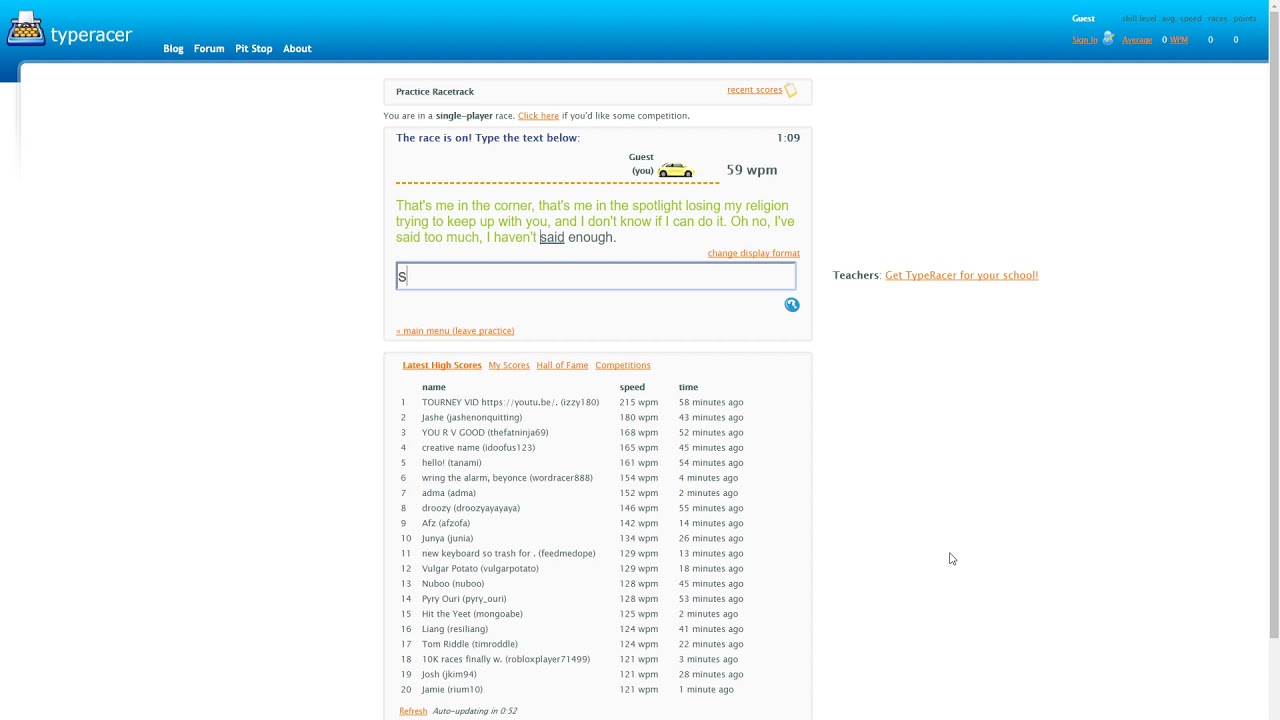**Detailed Caption:**

This image appears to be a screenshot from a website offering a typing teaching program. The design features a notable amount of empty space with small, centered text. At the top of the screen, a blue horizontal band spans the width of the page. In the left-hand corner of this band, a typewriter logo is visible, alongside the text "Type Acer," followed by navigational links labeled "blog," "forum," and "pitch shop." The right side of the blue band contains blurry orange links, with "guest" being the only partially readable word.

Centered below the blue band, the page header displays options like "practice race track," "recent scores," and "you're a single player race." Below this, there is a notable prompt suggesting users can "click here if you'd like some competition." The main section encourages users to engage in a typing challenge, instructing: "The race is on, type the text below." The prompt's text is sourced from the song "Losing My Religion" by R.E.M.: "That's me in the corner, that's me in the spotlight, losing my religion, trying to keep up with you. I don't know if I can do it. Oh no, I've said too much. I haven't said enough."

While engaging in the task, a small car icon symbolizes progress, and the achieved speed, displayed as "59 words per minute," suggests user performance. Beneath this interactive section, there is a comprehensive list, delineated into categories: "latest high scores," "my scores," "hall of fame," and "competitions." The list highlights names such as "journey," "vid," "YouTube video," "Josh," "creative name," "hello," and "Tanani," alongside their respective typing speeds. High scores range from 121 to an impressive 215 words per minute. Additionally, the list features embedded YouTube video links and an option to refresh the list at the bottom.